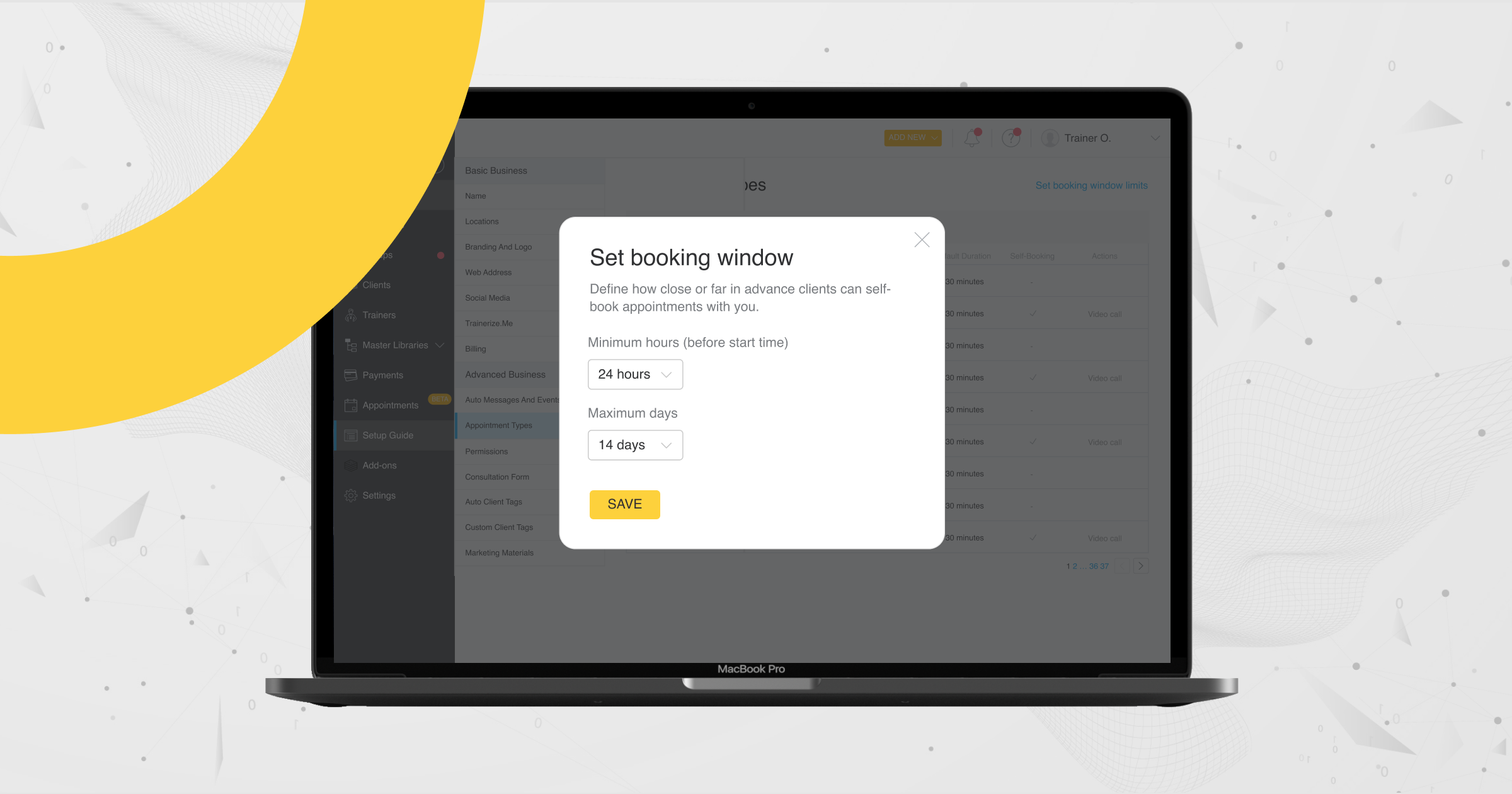The image depicts a silver MacBook Pro laptop open on a desk. The laptop screen showcases a busy interface with black bezels framing it. There is a prominent yellow rectangle on the screen that reads, "I'm New," indicating a notification or alert from an app or software.

In the background, the interface displays various tabs and sections, including "Clients," "Trainers," "Master Libraries," "Payments," "Appointments," and "Setup Guide." It also shows additional settings such as "Add-On Settings," "Basic Business" (with subsections including name, locations, branding, logo, web address, and social media), and "Trainer Resume."

Further details on the screen mention "Billing," "Advanced Business," and a series of how-to guides covering messages, events, appointment times, permissions, consultation form, and model client tags. The "Customer Logo Tags" and a "Center" option are also visible.

Additionally, there are settings instructions for "Set Booking Window," including parameters for defining how close or far in advance clients can schedule appointments, with settings like "Minimum Hours (before start time: 24 hours)" and "Maximum Days: 14 days."

The yellow rectangle's presence adds a focal point to the administrative and booking system presented on the screen, creating a vivid and informative narrative about the software's capabilities and interface.